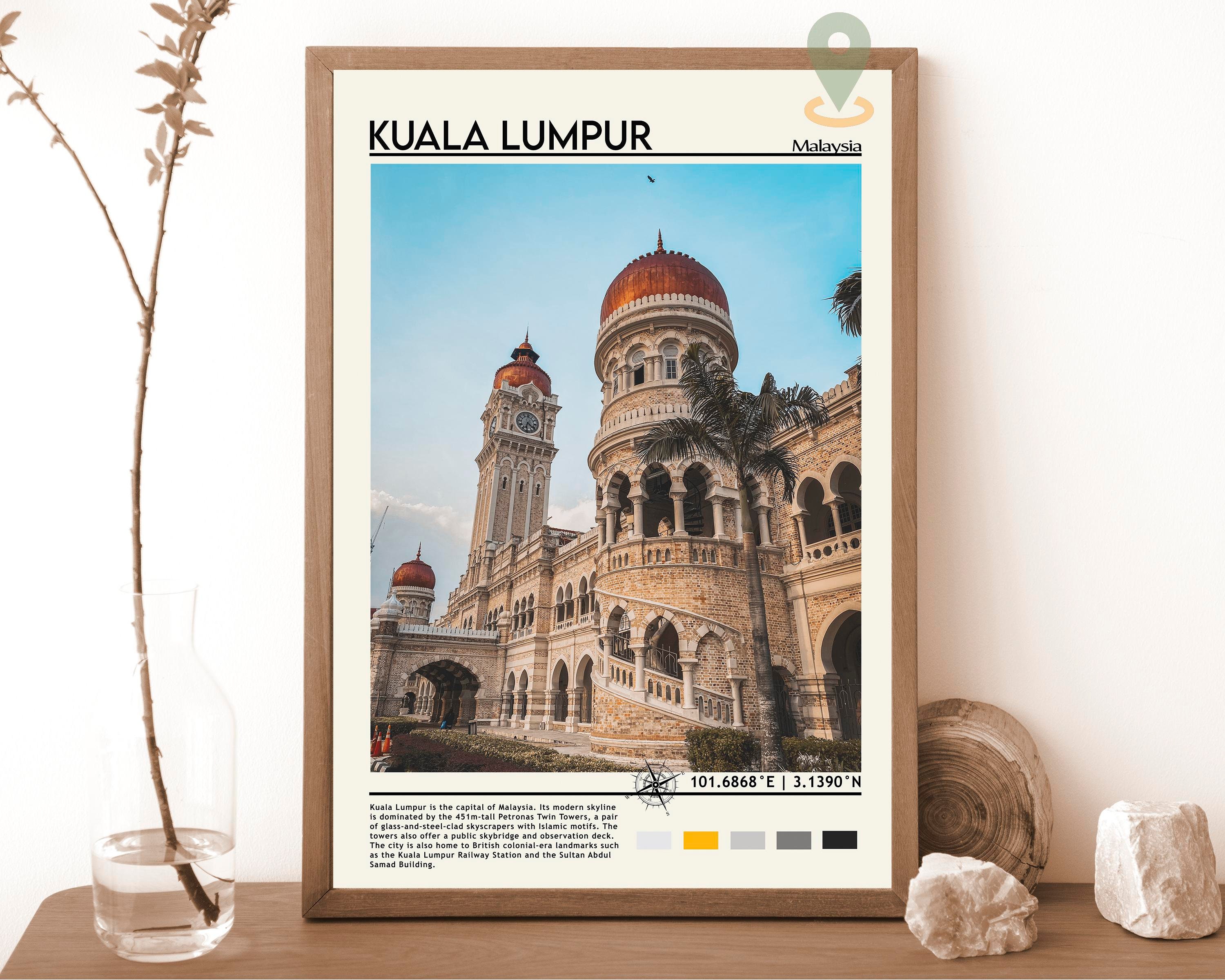The photograph captures a detailed composition centered on a framed image titled "Kuala Lumpur, Malaysia." The artwork, encapsulated in a medium brown wooden frame, features a vivid color photograph of an ornate building with domed towers set against a clear blue sky, exemplifying Malaysian architecture. The bottom left of the image includes unreadable text, and the lower right bears readable coordinates: 101.6868 degrees east and 3.1390 degrees north. Below these coordinates are five rectangles in varying shades: white or off-white, yellow, light gray, dark gray, and black. A compass rose is positioned between the picture and the rectangles. Intriguingly, a semi-transparent map logo in the upper right corner of the image displays the word "Malaysia" and overlaps the frame.

This framed art piece is situated on a brown wooden desk. To the left of the frame, there is a clear jar half-filled with water, holding a single twig with a few small brown leaves. On the right side of the desk lies a small piece of wood accompanied by two different kinds of small rocks. The background features a plain white wall, making the elements on the desk stand out prominently. The overall color theme leans towards light brown and white, adding a harmonious blend to the composition.